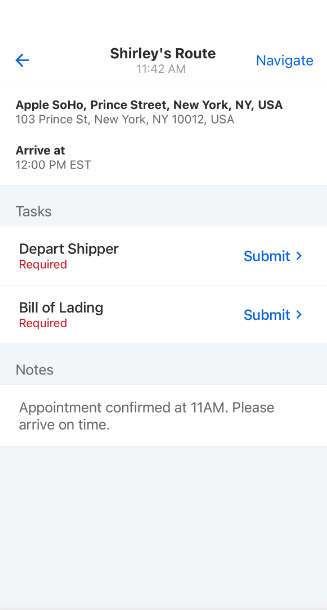The image has a white background with a detailed schedule layout. In the upper left corner, there is a blue left arrow. Centered and above a gray timestamp of "11:42 AM," there is the text "Shirley's Routine" in black. On the right side, the word "Navigate" is displayed in blue.

Below that, there is a list of tasks organized in a structured format:

1. **Apple Soho**: 103 Prince Street, New York, NY 10012, USA. The arrival time is set for 12 PM Eastern Standard Time.
   
   On a gray bar, detailed tasks are delineated:
   - "Depart Shipper" (in a block format).
   - The word "Required" is highlighted in red on the right, followed by "Submit" in blue and a blue right arrow.

2. **Bill of Lading**: Listed in black text with "Required" in red below it on the right, accompanied by "Submit" in blue and a blue right arrow.

A gray strip below these details marks the section titled "Notes." Underneath, on a white background with gray font, it states: "Appointment confirmed at 11 AM. Please arrive on time."

There are two inches of gray space at the bottom, possibly for additional information or notes.

There is one typo toward the end of the image, where "Shirley's Route" is misspelled as "RUTE."